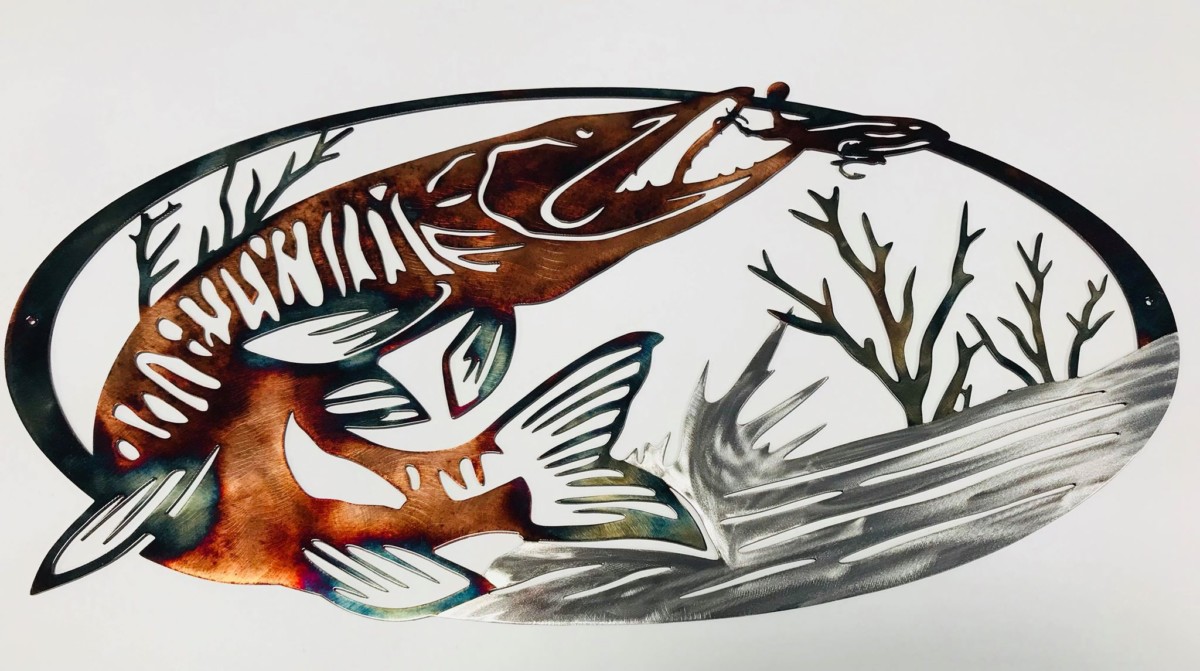This detailed, metallic decorative art piece, set against a white background, intricately depicts a dynamic underwater scene. The centerpiece is a twisting barracuda fish, characterized by its brown body with orange and black hues particularly concentrated on its lower sections. The fins and tail of the fish display a spectrum of green-blue and rainbowish colors, adding a vibrant contrast. The fish is captured mid-leap, arching in a U-turn as it appears ready to catch a smaller black fish or possibly a frog, evocative of a predatory pursuit.

Surrounding the fish, the artwork includes representations of grayish-black colored water, enhanced by metal foliage and coral structures on the right side. The coral varies in size, with a prominent, larger tree-like structure among them. The entire creation is formed within an oval frame, with certain areas intentionally left as hollow spaces, adding an intricate lattice-like quality to the piece. This elaborate sculpture, with its textured metalwork and vivid color contrasts, is beautifully framed within a white background, possibly hanging on a wall as an ornamental display.